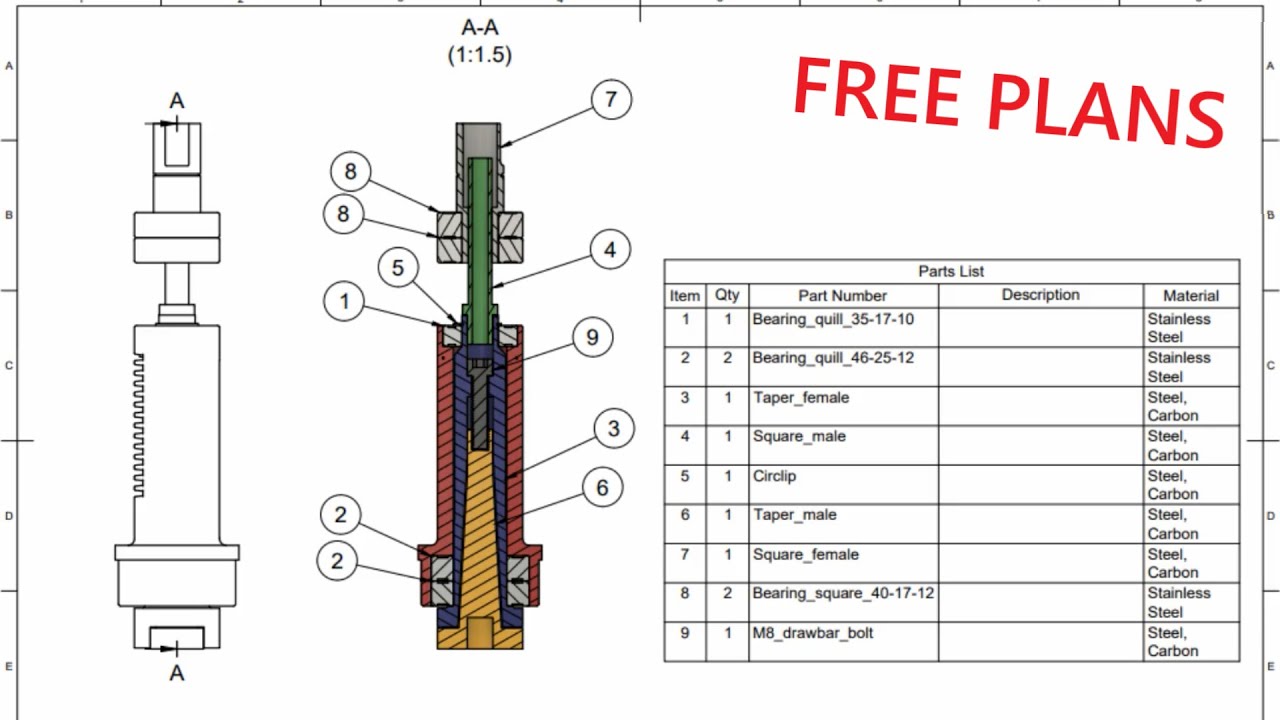The image is a detailed mechanical diagram on a white background, featuring both a black and white sketch and a colored drawing of a device resembling a spark plug. At the top right, bold red capital letters proclaim "FREE PLANS." The first depiction is a straightforward black and white outline, accompanied by a more intricate colored version that highlights different parts in green, red, yellow, and gray. Numbers from 1 to 8, circled and connected by lines, correspond to various parts of the device. These numbers are further explained in an included table, which lists part numbers, descriptions, materials, items, and quantities. The parts list identifies materials like carbon steel and stainless steel, with one example entry reading "bearing quill" along with its respective details. The ratio notation "AA, 1:1:5" is also included, contributing to the meticulous level of detail presented in this technical drawing.